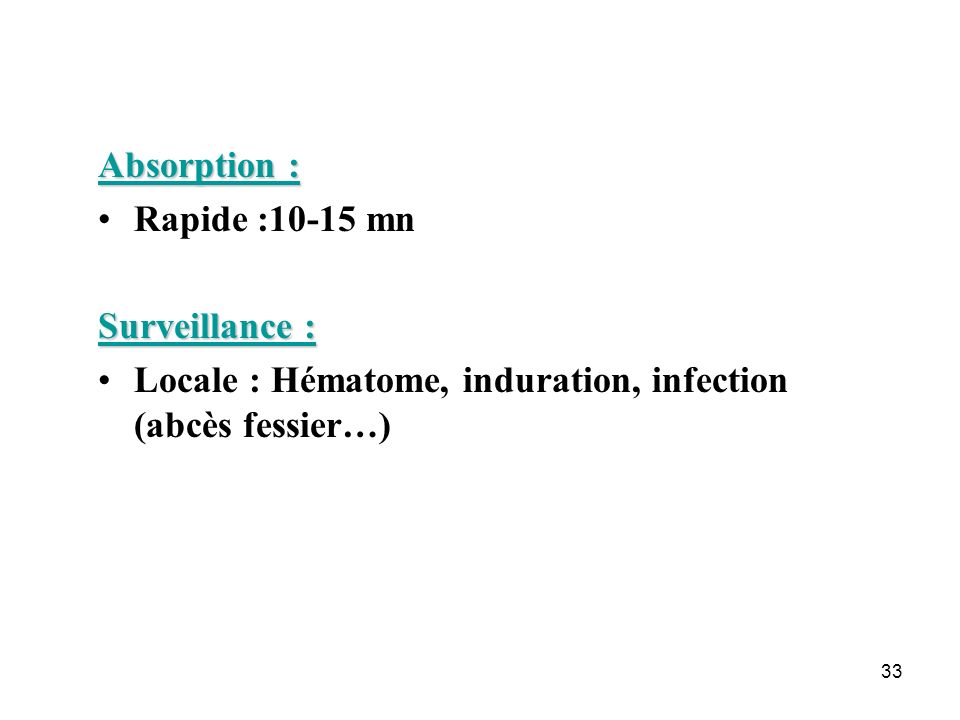The image features text with a predominantly white background, organized as if it were a page from a textbook or medical instruction manual, possibly related to pharmaceuticals. At the top, the word "Absorption" is underlined and formatted in blue text. Beneath this header is a radio button followed by the text "Rapid: 10 to 15 mm". Following this section, the word "Surveillance" appears, also underlined and in blue. Below it is another radio button with the text "Locale: Hematone, Induration, Infection (Abscess Facil)". In the bottom right corner of the image, the number "33" is displayed, likely indicating the page number.